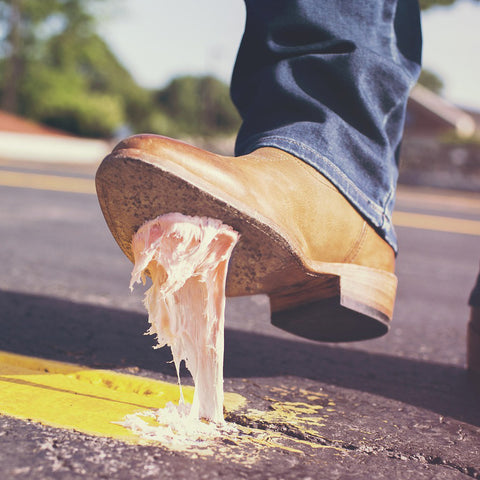This close-up, semi-realistic image depicts a person, presumably a man, who has inadvertently stepped on a large, fluffy piece of pink chewing gum on a black asphalt road marked with a yellow divider line. The man is lifting his foot, revealing the gum stretched between the roadway and the sole of his tan leather cowboy boot. The boot is worn and slightly scuffed, with a wooden heel and detailed stitching where the sole meets the upper part. He is dressed in dark blue boot-cut jeans that partly cover the boot. The gum, likely heated by the sun, is sticky and vividly pink, forming thick, stringy strands from the street to the bottom of the boot. The background, although blurred, shows more of the road, green trees, and the silhouette of a house in the top right corner, emphasizing the main focus on the unfortunate encounter with the gum.